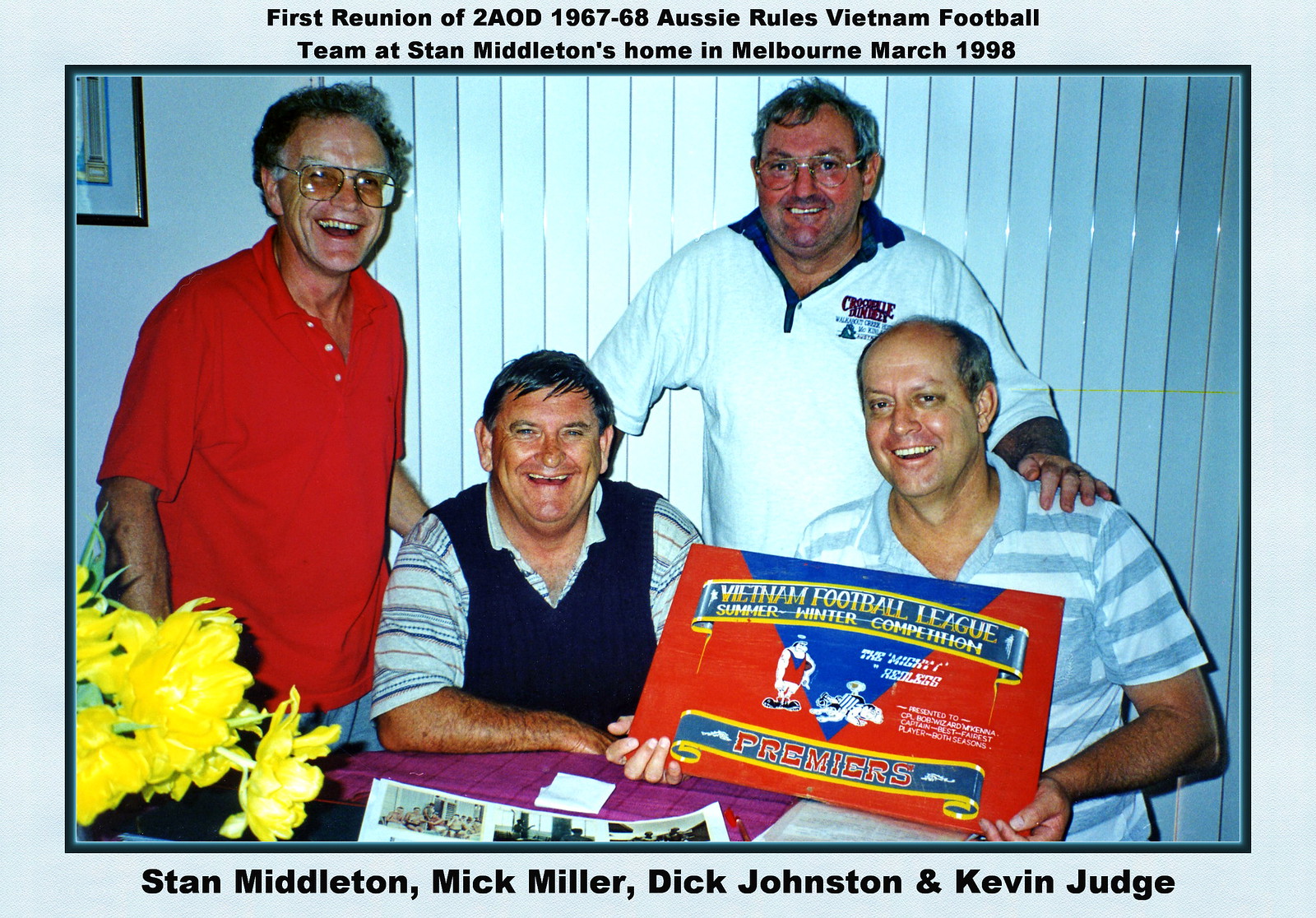This is a horizontally aligned, rectangular photograph bordered by a light blue background and a dark blue frame. Above the picture, black text reads, "First Reunion of 2AOD 1967-68, Aussie Rules Vietnam Football Team, at Stan Middleton's home in Melbourne, March 1998." The bottom caption names the four men in the image: Stan Middleton, Mick Miller, Dick Johnson, and Kevin Judge.

The four men, who appear to be retired members of the Aussie Rules Vietnam Football Team, are arranged with two standing and two seated in what looks like a living room. Behind them, white vertical blinds and a white wall adorned with a painting are visible. In the front, a small table holds a decorative arrangement of yellow flowers.

From left to right: the man on the left is wearing a red short-sleeve polo shirt and large glasses. He has curly, short, grayish-brown hair and is smiling broadly with his teeth showing. Sitting to his left, another man is wearing a blue sweater vest over a striped t-shirt. He also has short, gray and black hair and is smiling widely. Standing behind him is a man in a white polo shirt with a blue collar. He has glasses, short grayish-brown hair, and his left hand rests on the shoulder of the man seated at the far right. This man has a gray and white striped polo shirt, is bald on top with grayish-brown hair on the sides, and is smiling broadly while holding a red sign that reads, "Vietnam Football League Summer Winter Competition," with the word "Premieres" at the bottom.